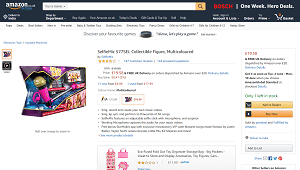This image shows a screenshot of Amazon search results. The primary product appears to be a pink microphone with a gray top, which resembles the protective grille commonly found on microphones. The handle is pink, and the product is depicted in approximately a three-quarter view. The packaging features pink and purple text, but the details are difficult to discern. The brand name looks like "BOSCH" in red letters. There is also a banner stating "One Week More Deals."

The usual Amazon interface elements are visible, including star ratings and various user options. However, the text is too small to read clearly. On the right side of the image, there's a price displayed in red, accompanied by buttons for adding the item to the cart or favorites, and a "Buy Now" button in orange.

Below the main product, there is a section for recommended products. Among these, one item seems to be a pink bag or perhaps a makeup kit targeted at children. Specific details, such as prices and exact product descriptions, are illegible due to the small text size.